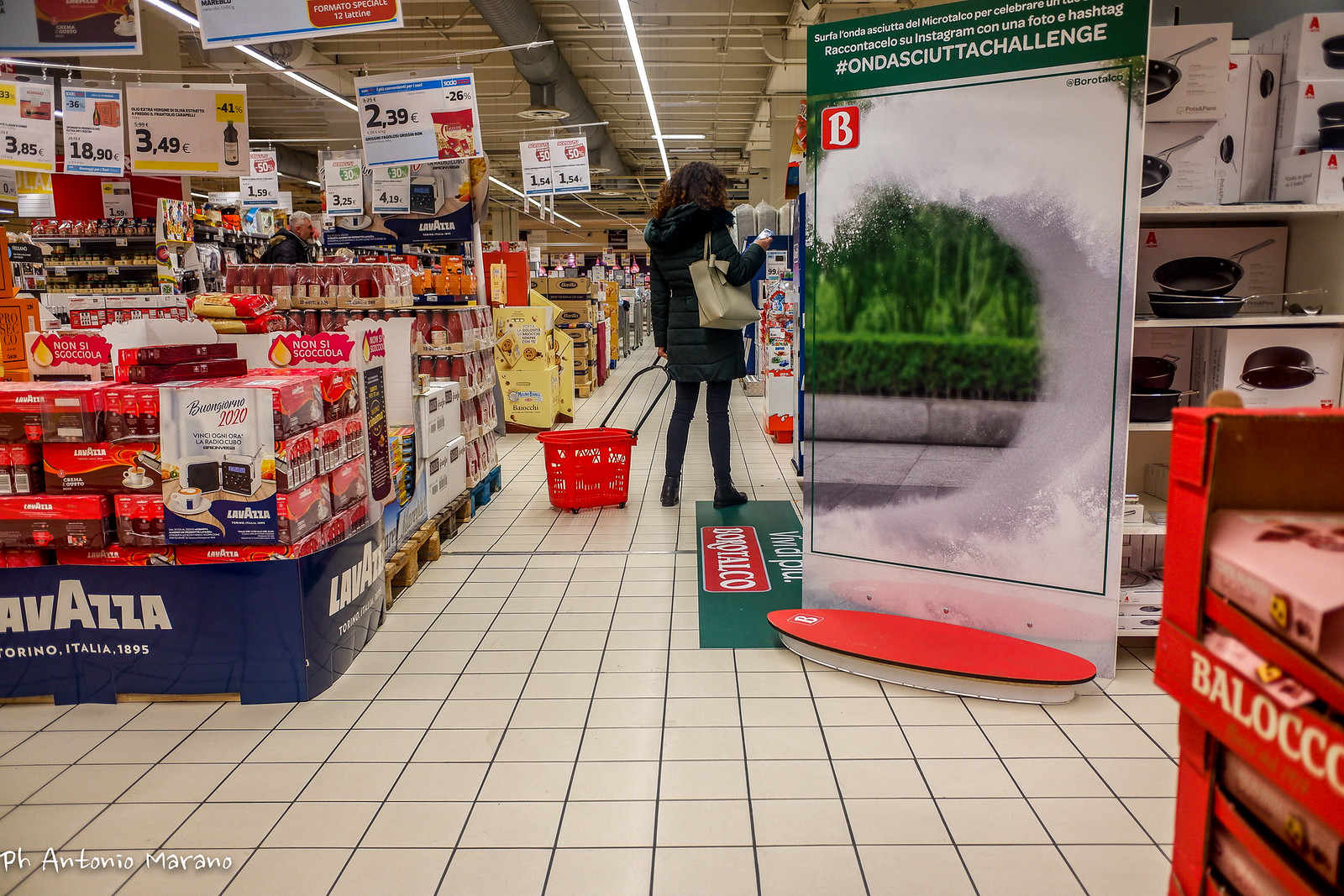Inside a spacious grocery store with a white tile floor, a woman is centrally positioned in the main aisle, partially facing away from the camera. She has dark, curly hair cascading down her back and is dressed in a long, dark coat paired with black tights and black shoes. Over her shoulder, she carries a cream-colored purse, and she pulls along a small red shopping basket. The aisle is flanked on the left by pallets stacked with diverse food items, including one with drinking water, and on the right, shelves display pots, pans, and various boxes. Above, advertisements including prices are prominently displayed; all are listed in euros, suggesting a European location, likely Spain or Italy. The background reveals another shopper, an older man with grey hair. Noteworthy signs include a large one in the middle of the aisle with an outdoor image and the phrase "Onda Skuitt Challenge," and in the bottom left-hand corner of the image, the name "P.H. Antonio Marano" is visible. The woman appears focused on reading the packaging of a product.